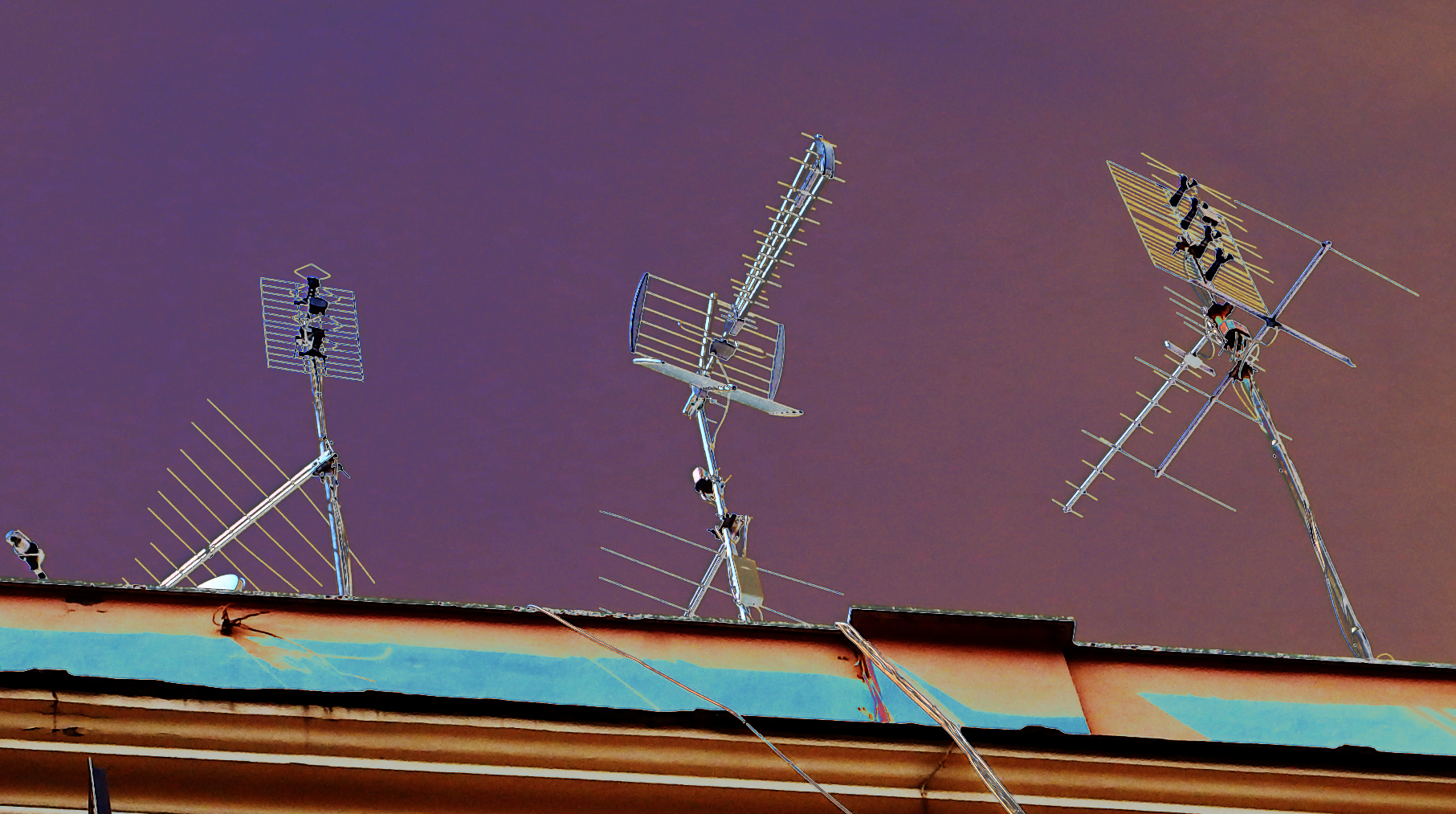In this surreal piece of digital art, the scene is viewed from the ground, looking up at a rooftop framed by a striking, gradient sky that transitions from dark purple on the left to a copper brown on the right. At the very bottom of the image, the edge of a roof is visible, bordered by a band that features both yellow and blueish hues. Atop the roof, there are three intricate antennas. 

The leftmost antenna, constructed of silver metal, features a triangular section with through-lines and a square shape at the top adorned with zigzag patterns. The middle antenna appears slimmer and includes a rectangular shape with a similar zigzag pattern, connected to a long, slender arm with several lines. The rightmost and largest antenna boasts a square shape on top, supported by a metal pole, and an elaborate array of interconnected lines and arms.

Scattered across the rooftop, which is painted in shades of greenish-blue and tan, are various cables and wires that snake their way to the antennas. The juxtaposition of the metallic structures against the vibrant, color-shifting sky creates an otherworldly atmosphere.